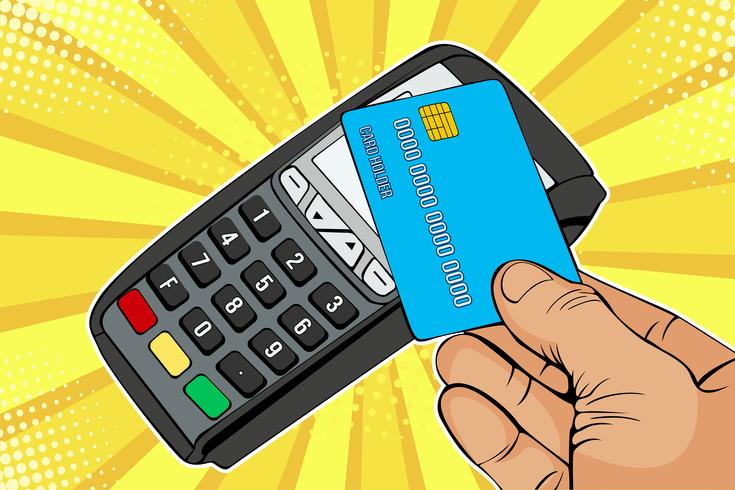The image is a cartoon-style, clipart graphic reminiscent of Marvel comic book illustrations. It features a light-skinned hand holding a blue credit card with a gold chip and white numbers displaying all zeros. The card, labeled "CARDHOLDER" in white letters, is positioned in the bottom right corner of the image. The hand is tapping the card against a black and white credit card reader. The device includes a number pad with buttons numbered 1 through 9, as well as a sequence of three buttons in red, yellow, and green beneath it. Above the number pad, there are up and down arrows. The background of the image is a vibrant, pinwheel-style pattern comprising various shades of yellow, with additional yellow rays and white dots enhancing the dynamic visual effect.